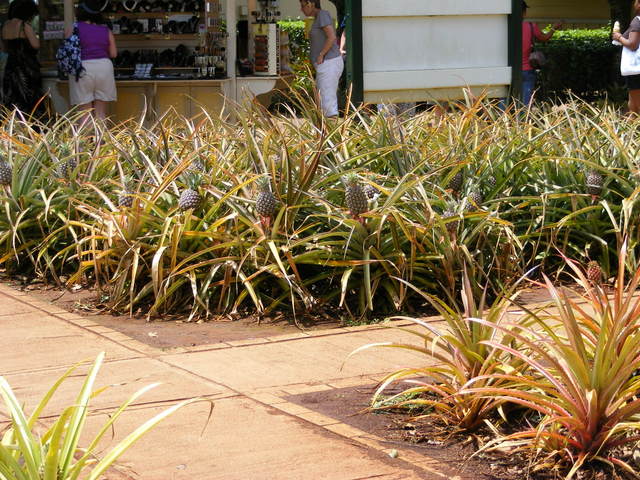The photo showcases a vibrant outdoor scene at a bustling retail area, captured during the day. In the foreground, intricately designed sidewalks intersect to form a cross pattern, separating rectangular garden patches. These gardens are planted with pineapple plants, characterized by their green and yellow leaves, some with brown tinges, and small pineapples at various stages of growth. The pineapples' crowns rise prominently from the dense foliage which spreads in multiple directions. Framing the scene is a display of black planters for additional flowers. In the background, a mix of pedestrians can be seen moving about, likely in a warm, possibly humid climate given their attire of shorts and short-sleeve shirts. Among them, a woman dressed in purple and white shorts, and another in white pants with a grey or silver top stand out, seemingly waiting in line at a jewelry kiosk or other storefront, contributing to the lively retail atmosphere. None of the people are looking towards the camera, emphasizing the garden and the pineapple plants as the primary focus of the image.